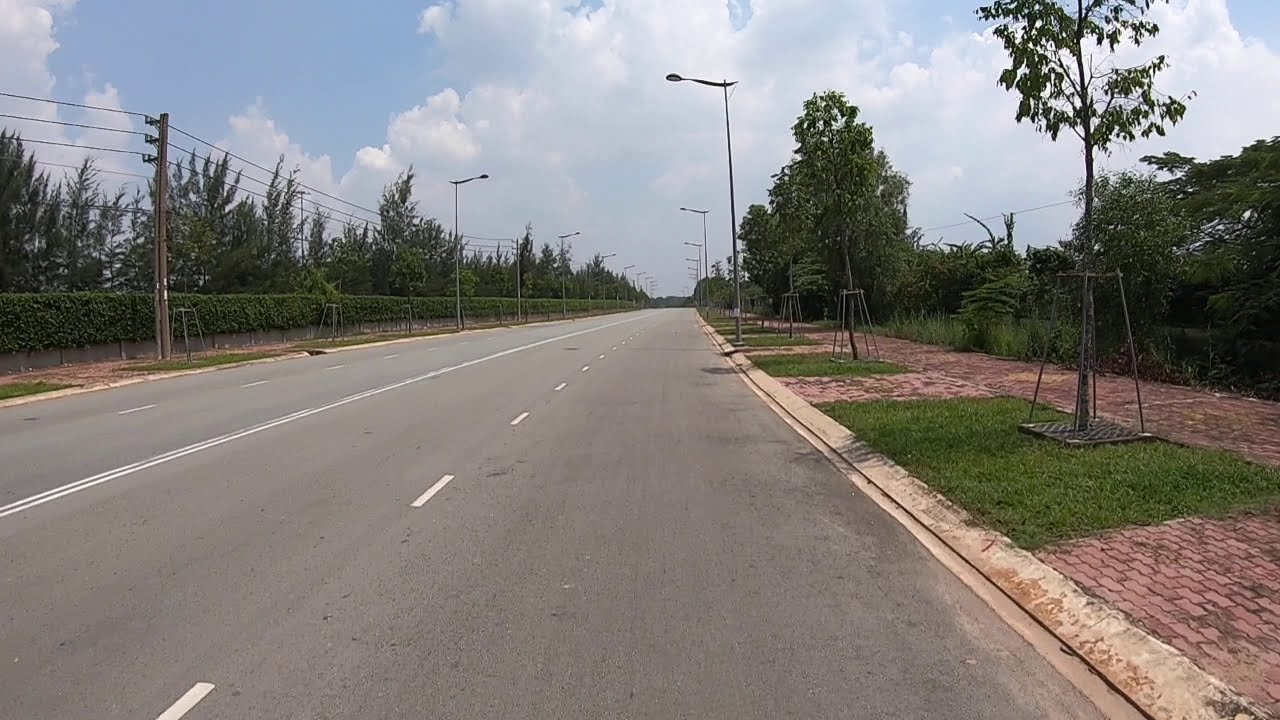The photograph depicts a long, straight, four-lane asphalt road that stretches into the distance. The camera perspective is from the furthest right lane, revealing three adjacent lanes separated by double white lines. Both sides of the road are bordered by wide brick sidewalks interspersed with alternating patches of grass. The grassy patches, which house young, slender trees supported by structures, create a pleasant rhythm along the sidewalks. These brick pathways lead to a denser area of greenery including tall bushes and more trees. Overhead, a network of power lines runs parallel to the street on the left, accompanied by numerous L-shaped streetlights that line both sides of the road. The sky overhead is a vibrant blue with large, fluffy white clouds, indicating a bright, sunny day. The overall tranquil atmosphere is enhanced by the lush patches of grass and clusters of trees on either side, with tree lines extending into the distance.